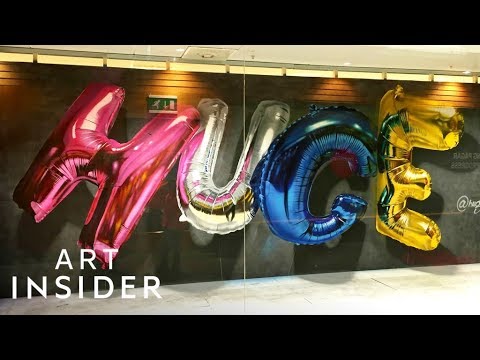The image showcases four giant mylar foil balloons in the shape of letters, vividly spelling out the word "HUGE." The balloons consist of a pink or red "H," a silver "U," a blue "G," and a gold "E." These eye-catching balloons are strongly illuminated by backlighting, giving them a shiny, reflective appearance. They appear to be either hung from a railing or placed against a wall, which might be part of a parking garage or a black marble-like surface. Positioned in the bottom left corner of the image, in white font, are the words "Art Insider." Additionally, there is a white floor resembling marble and the image is framed by two black bars. The overall setup suggests that this might be an advertisement for an art gallery or exhibit.